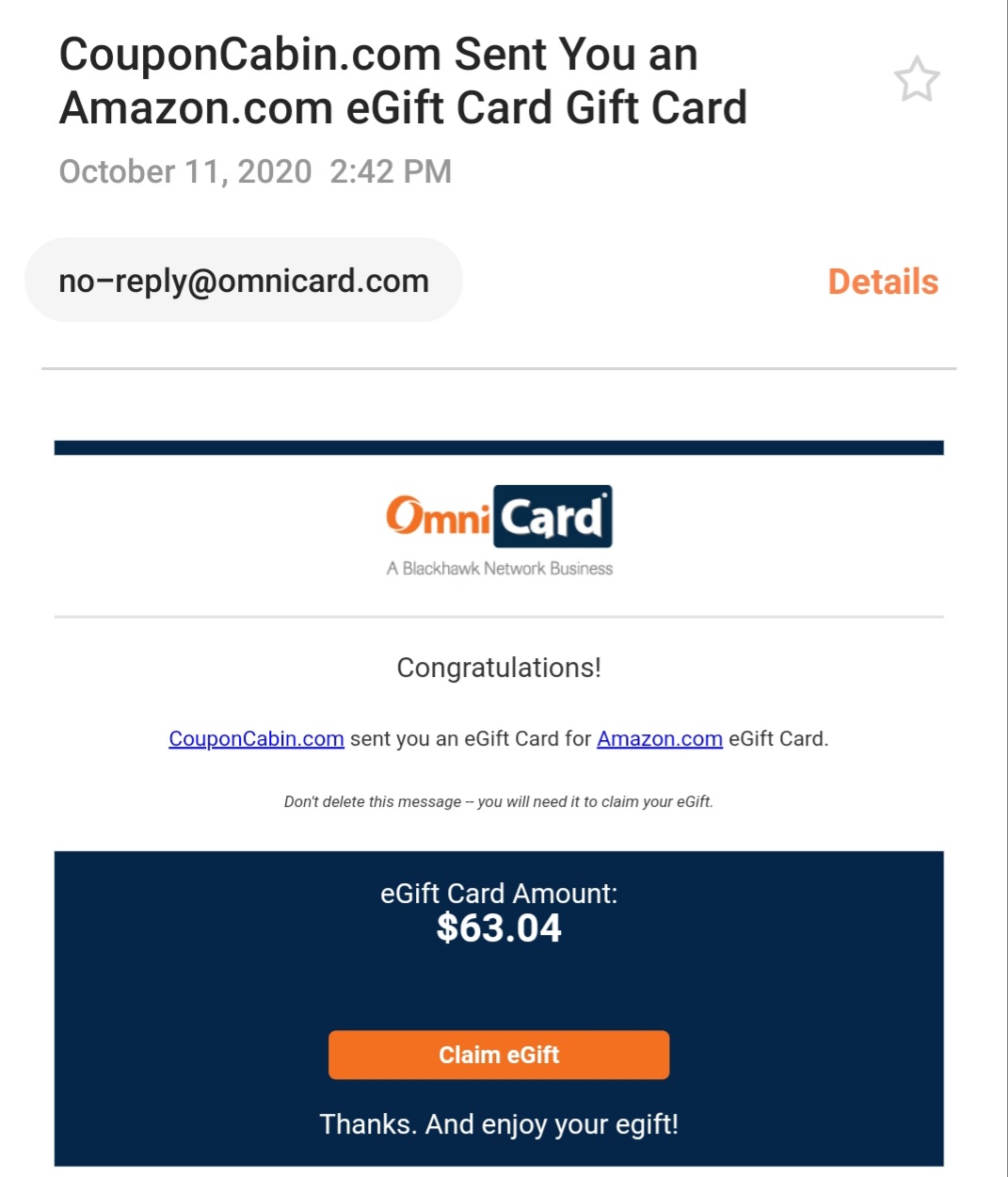Screenshot of an Email Notification for an Amazon.com E-Gift Card from CouponCabin.com

The image captures a screenshot of an email notification. At the very top, in prominent bold black text, it states: "couponcabin.com sent you an amazon.com e-gift card." To the right, there is a faded star with a gray outline. Below the bold text, the date is clearly indicated as "October 11th, 2020, 2:42 p.m."

Directly beneath the date, there's a text bubble with a light gray background containing black text that reads "no-reply@omnicard.com." To the right of this bubble, there is a large orange button labeled "Details."

The email also features the Omnicard logo, where the letter 'O' has distinctive splices. This logo is in orange, with "Omnicard" written in white text against a dark navy blue background. Below the Omnicard logo, it is noted that this is "A Blackhawk Network Business."

The body of the email begins with an enthusiastic congratulatory message: "Congratulations!" followed by, "Couponcabin.com sent you an e-gift card for Amazon e-gift card." Below this statement, there's a cautionary note in very small text: "Do not delete this message, you will need it to reclaim your e-gift."

Towards the bottom of the email, the amount of the e-gift card is specified as "$63.04." Lastly, there's a prominent orange box labeled "Claim E-Gift," inviting the recipient to redeem their card.